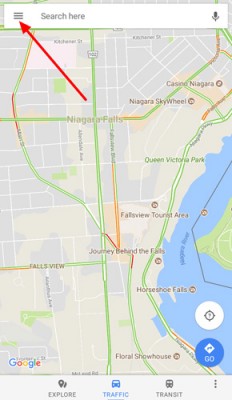The image depicts a map interface with several key features and landmarks. At the top, there is a search box with a "hamburger" menu icon on its left side, highlighted by a large red arrow. Within the search box, the text "Search here" along with a microphone icon are visible. The map itself displays roads marked in various colors—green, orange, and red—indicating different traffic conditions. There is a body of water on the right side of the map. Notable landmarks include Casino Niagara, Niagara Falls, Niagara Sky Wheel, Queen Victoria Park, Fairview Tourist Area, Journey Behind the Falls, Fallsview, Horseshoe Falls, and Floral Show House. The interface also shows the Google icon on the left and a blue "Go" button on the right. At the bottom of the screen, options labeled "Explore," "Traffic," and "Transit" are visible.